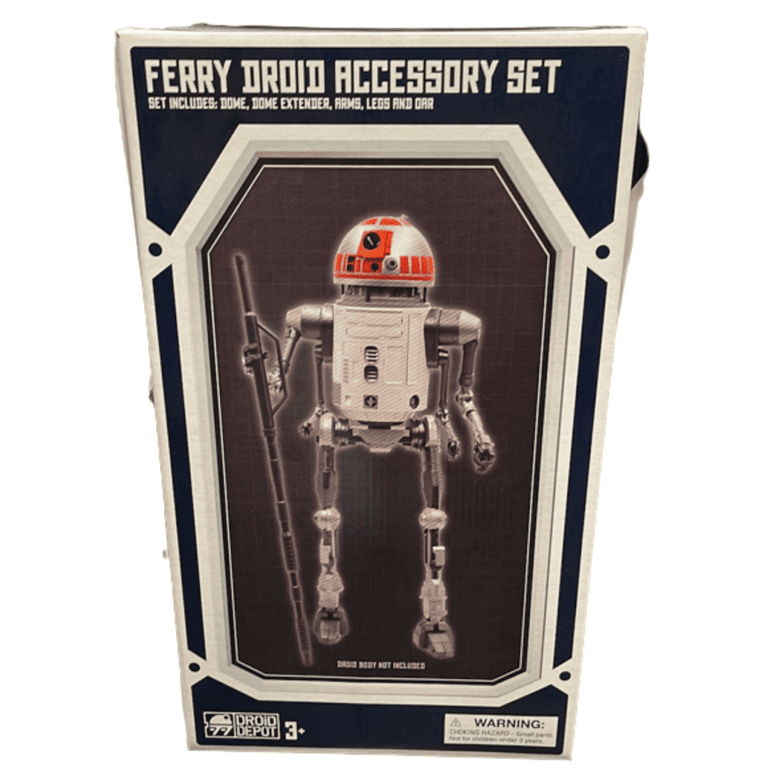The image is a vertically aligned rectangular photo showcasing a toy robot from the Star Wars universe against a white background. The box, primarily navy blue and perhaps black, is topped with the title "Fairy Droid Accessory Set" in bold white all-caps. Below the title, smaller white all-caps text lists the included items: "Dome, Dome Extender, Arms, Legs, and Ore." The featured robot resembles R2-D2, with a rounded head in gray and orange instead of blue, and a humanoid body with articulated arms and legs. One of its right arms holds a long, metal staff, described as an "ore." The lower left corner of the box displays the "Droid Depot" logo and text indicating it is suitable for ages "3 Plus." The lower right corner contains a white rectangular box with "WARNING" in black all-caps and finer print warning of a choking hazard due to small parts.